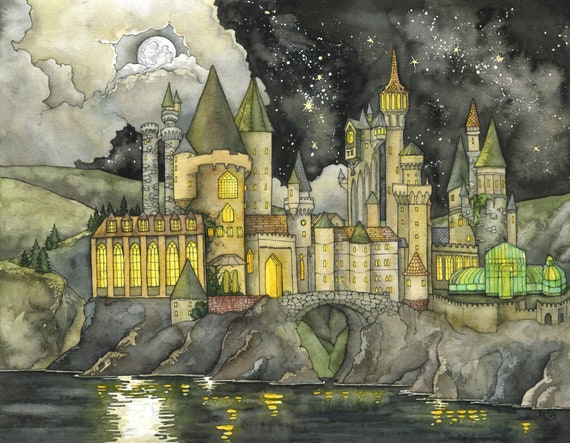This computer-animated painting depicts an expansive, enchanted castle perched on a massive gray mountain, flanked by rolling green hills and lush trees. The castle features many towers adorned with triangular domes and peaks, illuminated by bright yellow and amber lights streaming from numerous windows. A cement bridge spans a reflective body of water, creating a scenic moat that surrounds the hill. The night sky above is a captivating mix of black and gray hues, dotted with twinkling stars predominantly on the right side, and graced by thick white and gray clouds opening up to reveal a luminous gray moon. The overall atmosphere combines elements of marker, watercolor, and ink pen artistry, encapsulating a mystical and serene fantasy landscape.